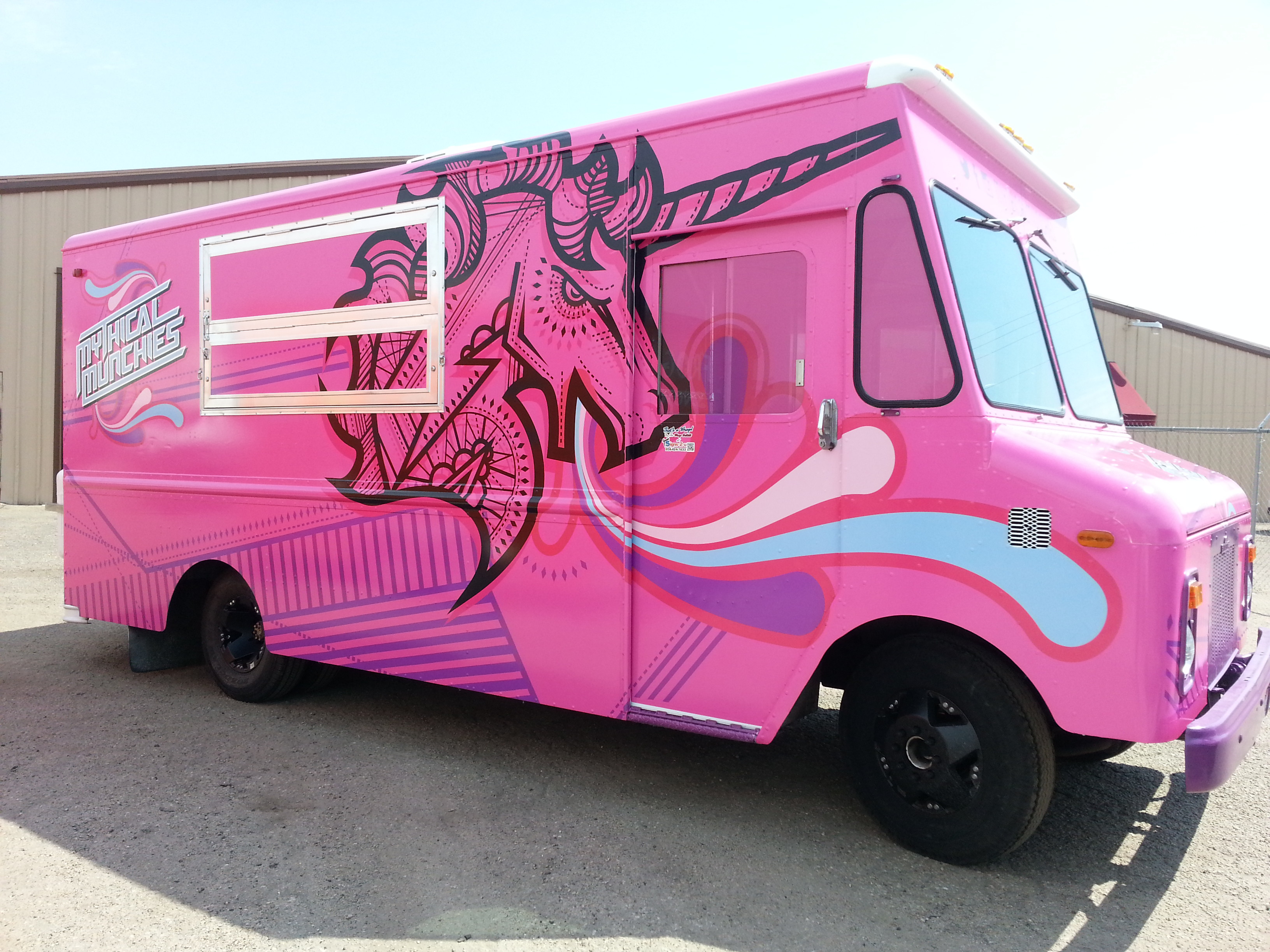This photograph features a brightly colored pink food truck named "Mythical Munchies" parked in front of a gray warehouse on a concrete surface. The truck, resembling a tall and long cargo van, is fully wrapped in vibrant hues of pink, purple, white, and light blue. Dominating its side is an intricate vector illustration of a black unicorn adorned with abstract, geometric, and tribal patterns. The unicorn design spans the length of the van, with its horn extending towards the front. The unicorn appears to be exhaling colorful, rounded streaks and swirls, further decorated with watery floral lines. Above the food serving window, which is currently closed, the name "Mythical Munchies" is prominently displayed, possibly the logo of the company. Additional geometric patterns in purple accentuate the food truck's vivid and fantastical theme. The front bumper of the truck is purple, and the top lights are white, adding to its whimsical appearance. The truck’s black tires rest on smooth concrete, completing the composition of this enchanting mobile eatery.